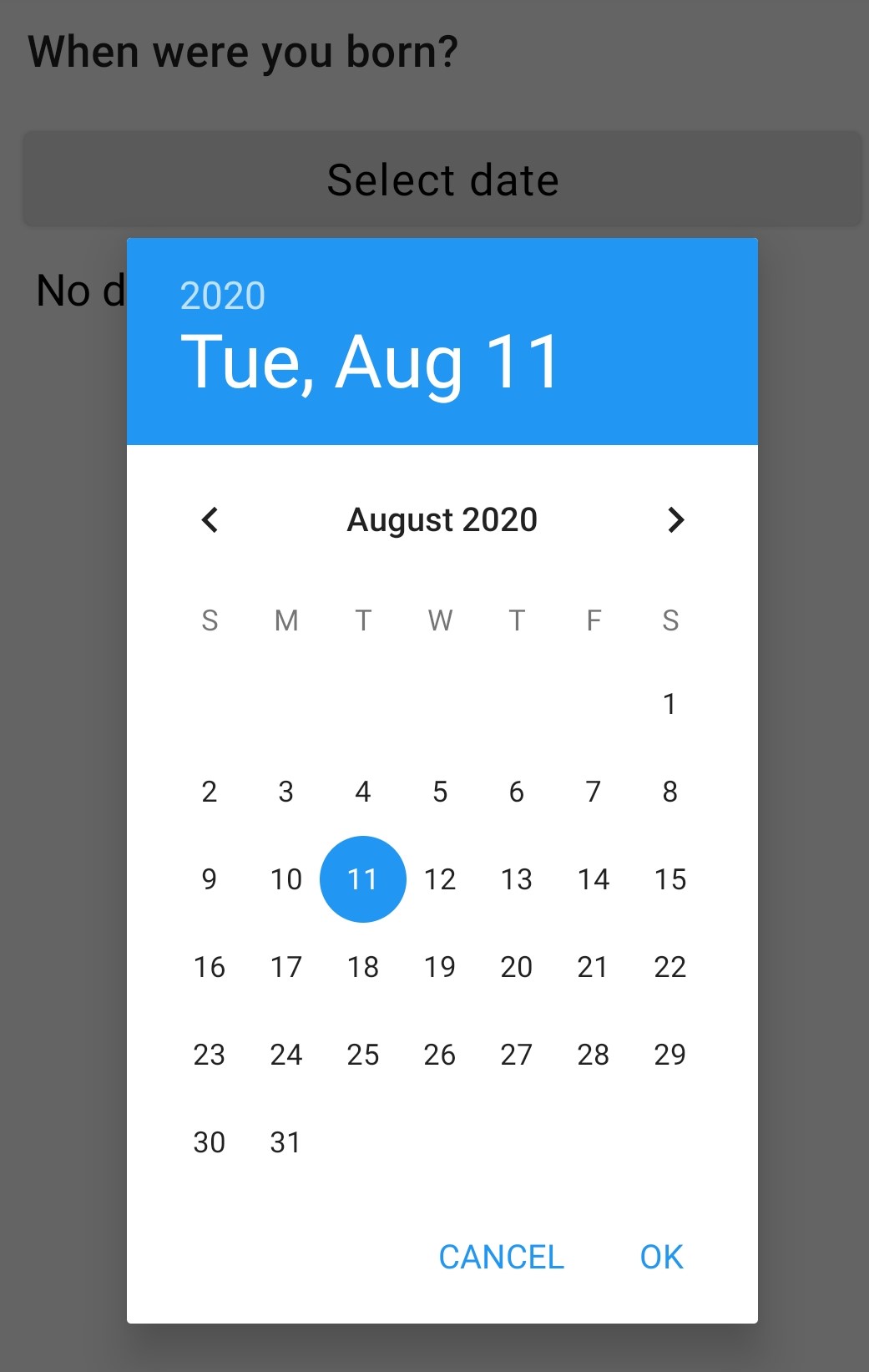The image shows a digital calendar interface from August 2020. The top of the calendar prominently displays the year "2020." Below this, in a larger white font, the day of the week "Tuesday" is highlighted, accompanied by the full date "TUE, Aug 11." The calendar itself has a white background with the month "August 2020" centered at the top in black text. Navigation arrows are visible on both sides of the month title, allowing users to switch between months.

The calendar days are arranged in a grid, with the days of the week abbreviated to single letters (S for Sunday through S for Saturday). The first day of the month, Saturday, August 1st, is marked with a blue circle around the date. At the bottom of the calendar, two buttons labeled "Cancel" and "OK" allow the user to either discard or confirm their selection. If the calendar is exited or canceled, the interface returns the user to the previously viewed page. The currently selected date is notated above a grayed-out section labeled "NoD," indicating no details are provided for the selected date.